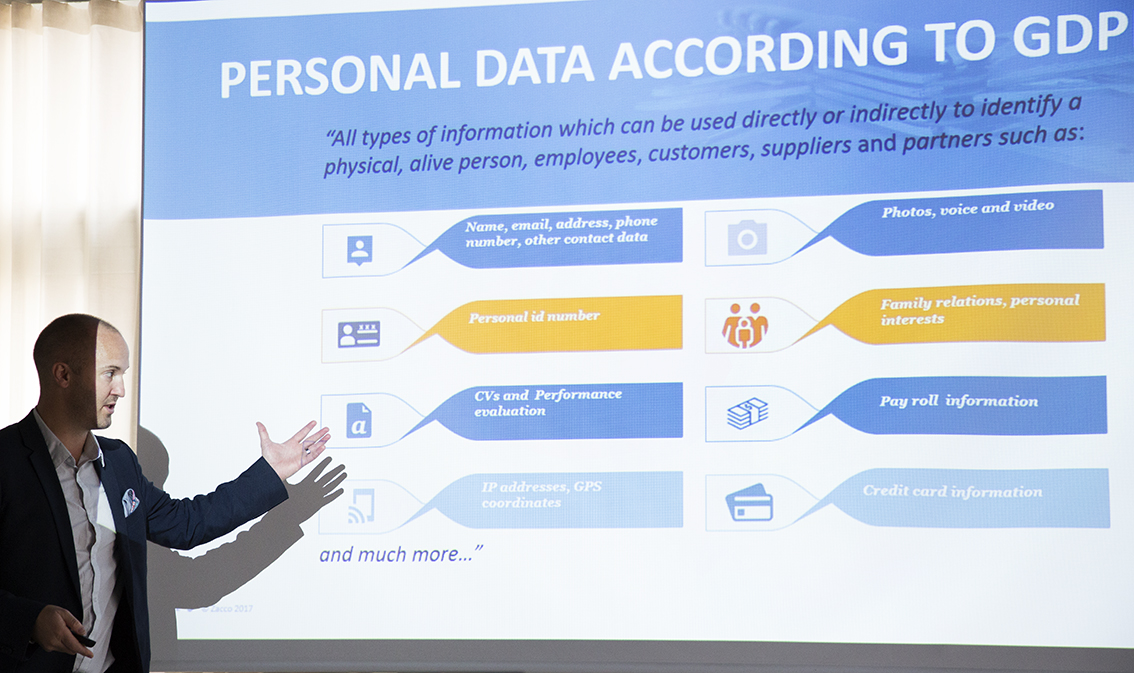The image captures a man, in his 40s, delivering a presentation. He is positioned at the bottom left of the frame, dressed in a dark blue suit jacket with an embossed design on the left side and a white button-up shirt. A wedding ring adorns his finger. The presenter, slightly bald, points with his left hand towards a large screen behind him. The screen, white with a blue strip at the top, prominently features the heading "Personal Data According to GDP" in white font over a blue background. Below this, in a darker blue font, the screen details various types of information that can be used directly or indirectly to identify a person, including employees, customers, suppliers, and partners. The listed data types include name, email address, phone number, other contact data, personal ID number, CVs and performance evaluations, IP addresses, GPS coordinates, photos, voice and video, family relations, personal interests, payroll information, credit card information, and more. Each item is accompanied by a corresponding icon—such as a camera for photos and video, a cartoon ID for personal ID numbers, and a stack of bills for payroll information—organizing the information in a visually engaging manner. The man’s engaged posture and gesture towards the detailed screen emphasize the comprehensive nature of the data presented.